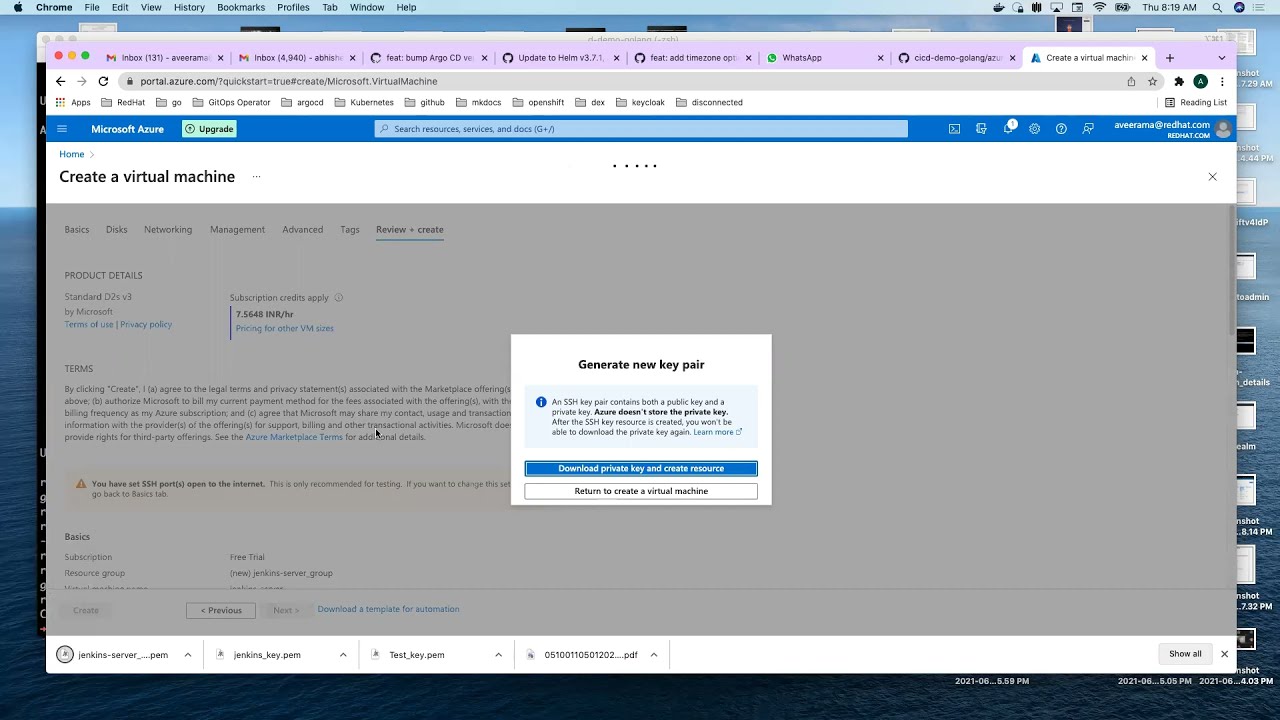This screenshot captures a section of the Microsoft Azure website interface. In the upper left-hand corner, there's a green "Upgrade" button. Below it, the navigation menu includes a home button and a highlighted option that reads "Create a Virtual Machine."

Further down, product details for a "Standard D2S V3" virtual machine by Microsoft are displayed, along with links to the "Terms of Use" and "Privacy Policy." Detailed terms are accessible directly underneath these links.

A prominent pop-up box titled "Generate New Key Pair" appears in the center of the screen. This box includes a blue information banner explaining that an SSH key pair consists of a public key and a private key, emphasizing that Azure does not store the private key post-creation; thus, it cannot be downloaded again. 

Beneath this explanation are two action buttons: "Download Private Key and Create Resource" and "Return to Create a Virtual Machine."

On the upper right-hand side, the user’s address is displayed as "avirama@redhat.com," with a reference to the "redhat.com" website directly below it.